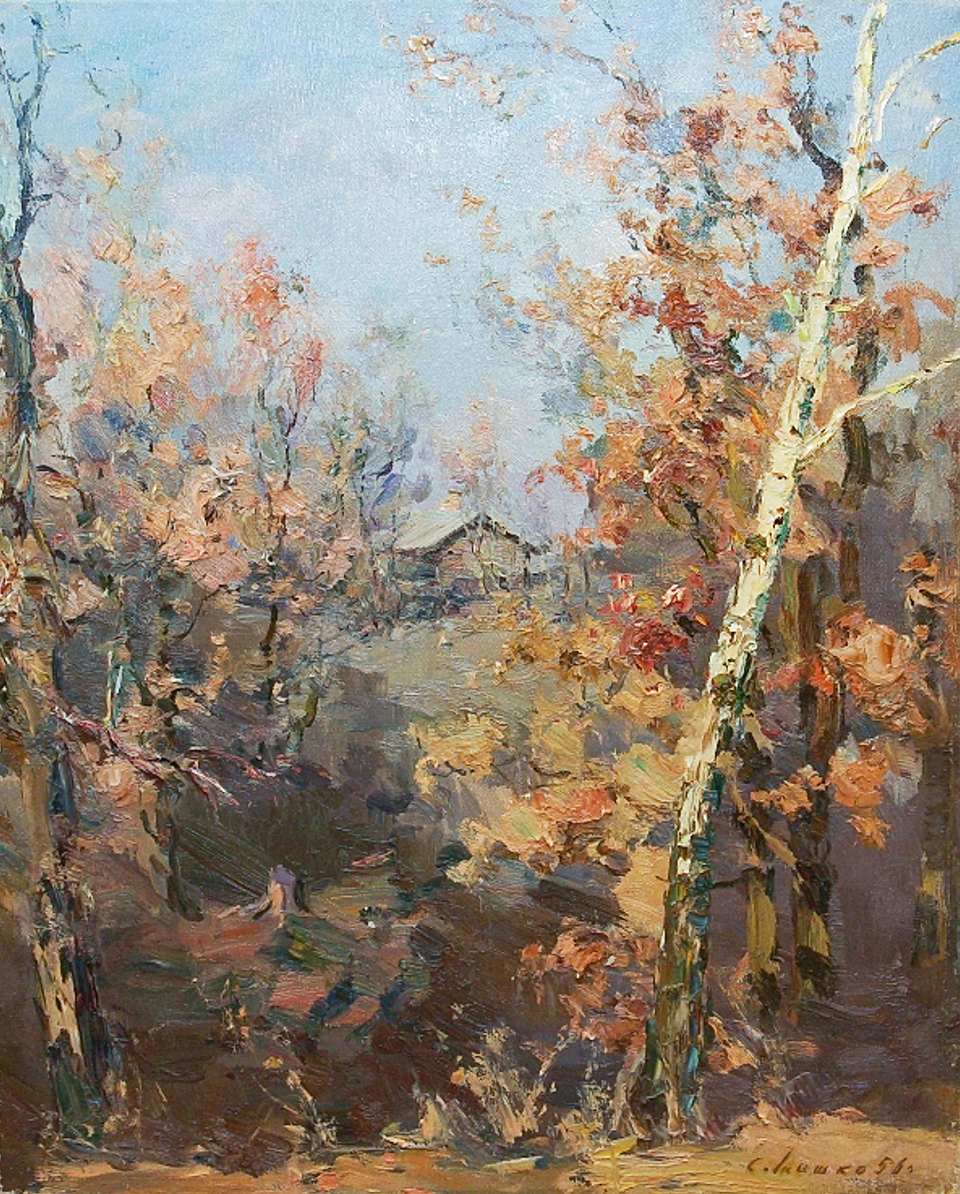This vibrant painting depicts a serene woodland scene bathed in the light of a clear blue sky. At the center of the composition, a small, cream-colored wooden house with a dark brown, triangular roof sits in the distance, offering a focal point amidst the tranquil surroundings. The foreground is rich with diverse plant life, including numerous trees adorned with fall foliage in hues of light orange, red, and yellow, while the ground beneath them is a muted brown. Among these trees, a prominent birch tree stands on the right side, distinctive with its white and green trunk. Scattered throughout are blooming pink flowers, adding bursts of color amidst the earthy tones of the landscape. The brushstrokes are vivid and expressive, with intentionally muddled boundaries that enhance the painterly effect. In the bottom right corner, a signature is present, suggesting the artist's name begins with a 'C', though it remains partially illegible. This detailed painting, oriented in portrait, captures the essence of an autumn day in the woods, exuding a sense of quiet beauty and timelessness.